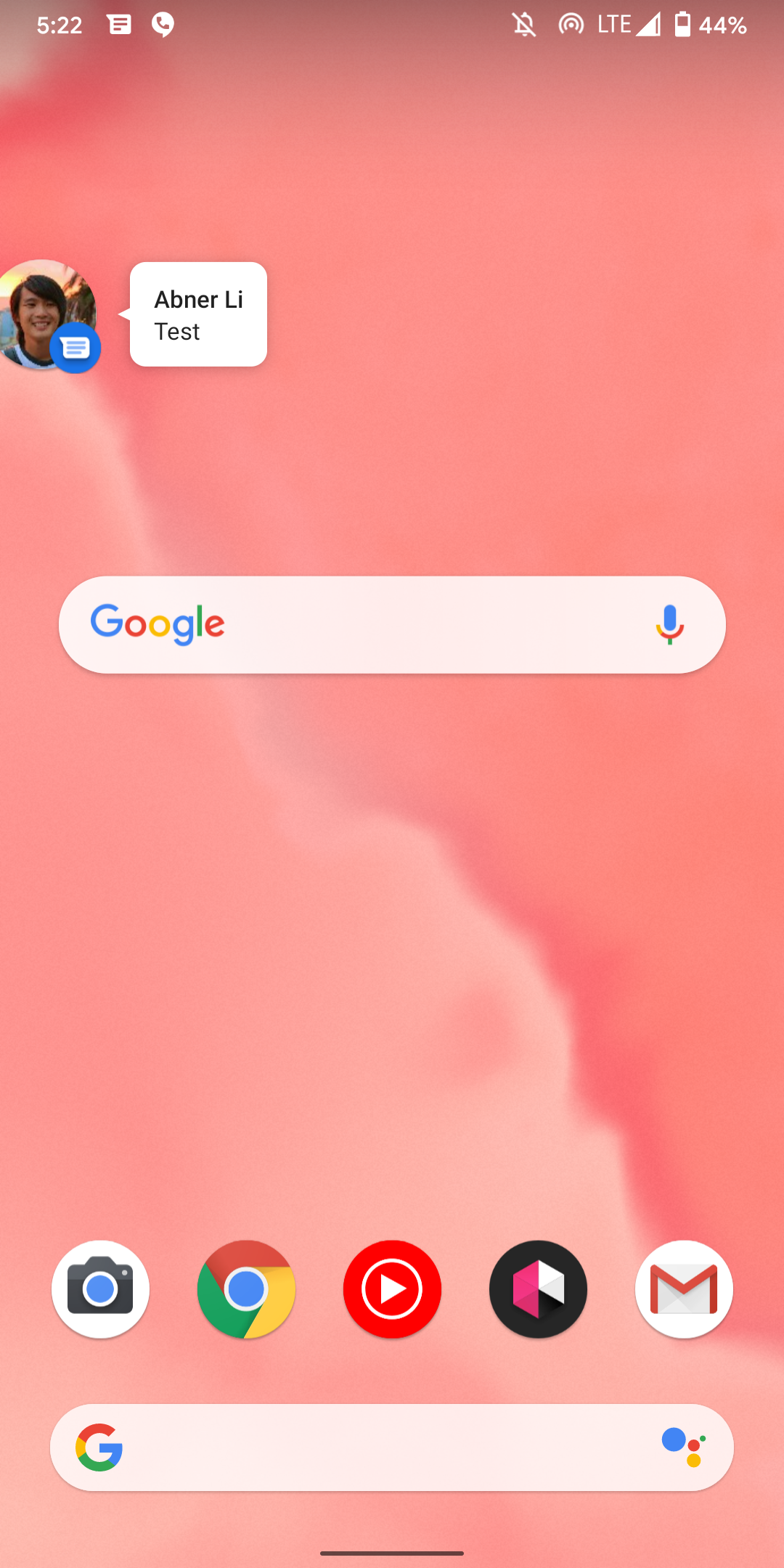This is a detailed screenshot of a cell phone home screen, featuring a background image in shades of salmon and light pink, resembling a close-up of a cloud against a pink sky. At the very top of the screen, a dark pink gradient overlays the background and integrates with various status icons. 

On the top left, the time is displayed as 5:22, followed by a chat symbol and a mobile signal indicator. To the right, there is a notification bell with a line through it, signifying silenced notifications. The signal strength bars indicate LTE connectivity, and the battery icon shows a 44% charge.

Positioned just below the top quarter of the screen is an oval-shaped Google search bar. The Google logo is displayed in its iconic full-color scheme (blue, red, yellow, blue, green, red), while a microphone symbol is located on the right side of the search bar.

At the bottom of the screen are five circular app icons arranged horizontally. From left to right, the first icon represents the camera, the second opens Google, the central icon with a white circle and play arrow likely opens YouTube, the fourth icon appears as a pink and white cube, and the fifth icon is for Gmail, depicted as a stylized "M" on an envelope within a white circle.

Beneath these icons, there is another search bar with a Google "G" logo on the left and a configuration of dots on the right side.

Between the central Google bar and the top of the screen, a message notification is visible on the left side. It features a circular contact photo of a young man with dark hair, accompanied by a blue message icon. Next to the photo is a white text box containing the sender's name, "Abner Lee," in bold, with the phrase "from Abner Lee" underneath.